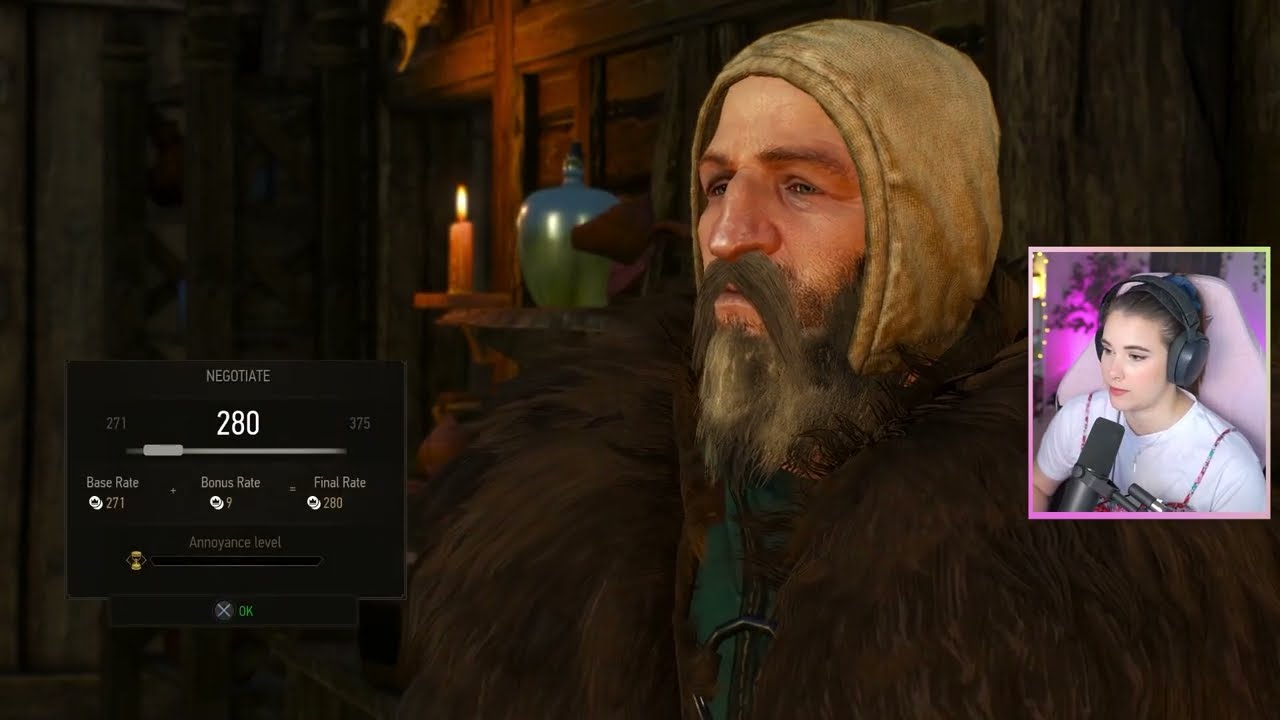The image is a very wide rectangular screenshot from a video game stream, featuring a detailed and vividly colored illustration of a tavern or old-fashioned house interior. The background showcases orangey-brown wood walls that turn gray towards the edges, adorned with a shelf, a burning candle, and a blue-green jug. The main focus is slightly to the right of center, depicting an older man who resembles a wizard or magician. He has a dark gray beard with lighter spots and wears a somewhat dirty tan hood along with an enormous brown fur coat. To the right, there is an inset window featuring a young woman, the game player, sitting in a pinkish chair with a light purple background. She is wearing a white t-shirt, headphones, and appears to be speaking into a microphone. Her hair is pulled back. The bottom left corner of the image includes game information with the word "negotiate" in white lettering above a strength bar indicating 280. The blend of video game illustration and real-life photography creates an engaging and immersive scene.